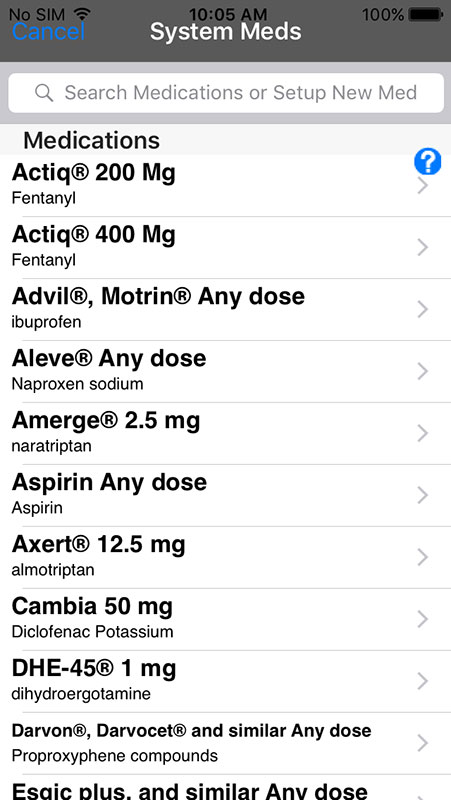This is a screenshot from a cell phone displaying a medication management app. At the top center of the screen, the time is shown as 10:03 AM. To the right, the battery icon indicates a full charge at 100%, while the top-left corner displays "No SIM."

Below the time, the label "System Meds" is prominently displayed in white text. To the left of this label, there is a blue "Cancel" button. Beneath this section, a search bar allows users to search for specific medications.

Further down, the background turns white with all text in black, heading with the word "Medications." It lists several medications along with their dosages:

1. **ACTIQ 200mg** - Fentanyl
2. **ACTIQ 400mg** - Fentanyl
3. **Advil/Morton** - Any dose, Ibuprofen
4. **Aleve** - Any dose
5. **Emerge 2.5mg** - Aspirin, Any dose
6. **Excerpt 12.5mg**
7. **Gambria 50mg**
8. **DHE** - Mg unspecified
9. **Darvin** - Any similar medication

This detailed view helps users track and manage their medications efficiently.